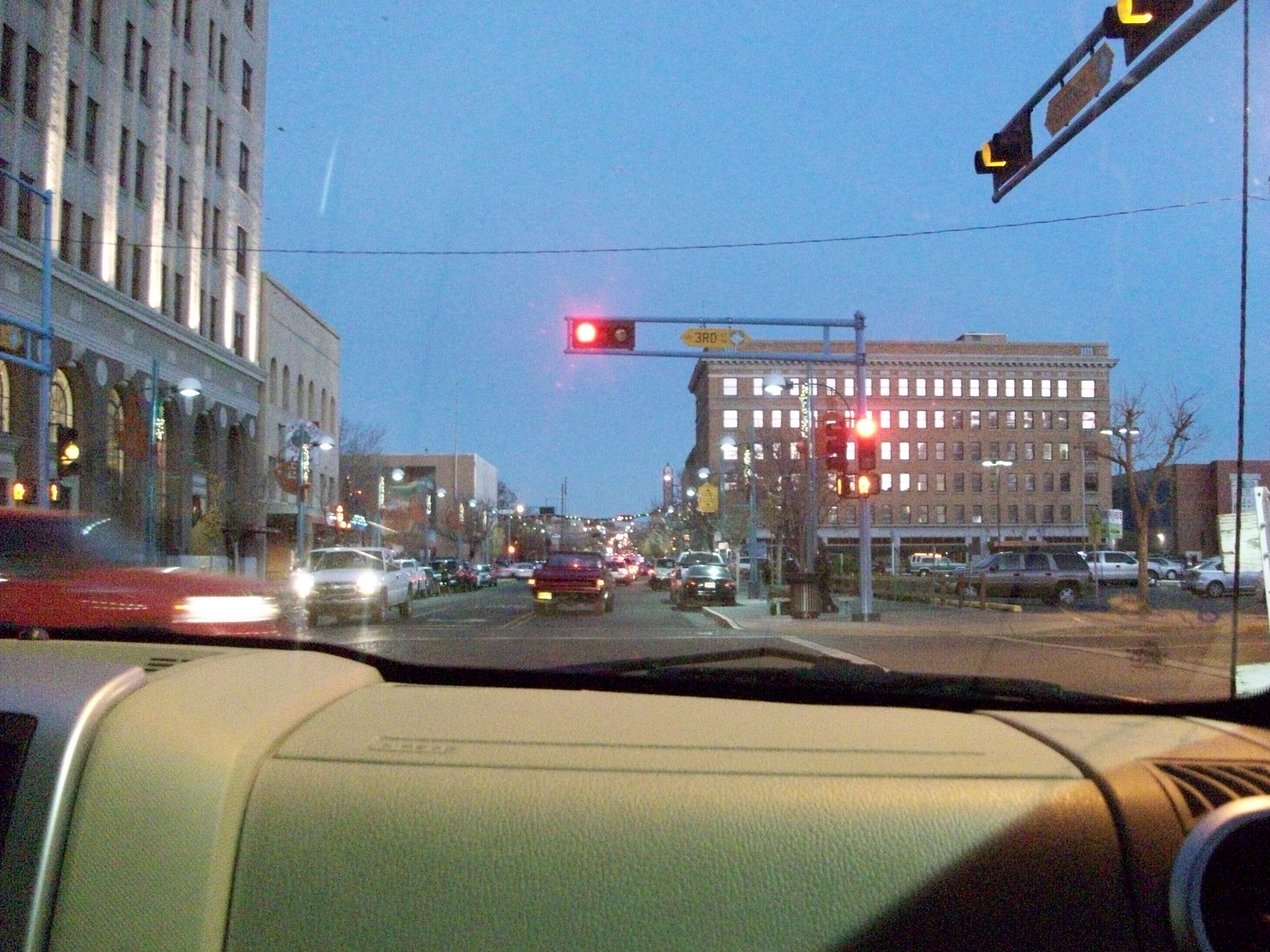The photograph captures an urban street scene from the perspective of a passenger seat in a car with a tan interior, accentuated by silver elements on the center console. A circular air freshener with a silver exterior and black center is attached to the vent. The center of the image is dominated by a red stoplight, indicating that the vehicle is halted at an intersection in the far right lane. The outside setting transitions towards dusk, with a grayish-blue sky dimming into night, casting long shadows. The urban environment features commercial buildings on both sides of the road. Notably, a large stone-walled building stands prominently on the left, and in the background, a tall brown building with many windows looms. The streets are busy, with a steady flow of traffic—headlights and taillights glowing brightly. A red car speeds past on the left, while a white car waits slightly ahead in the far left lane, and parked cars line a lot across the street to the right. The composition and the lighting collectively evoke the bustling yet serene transition from day to night in a cityscape.